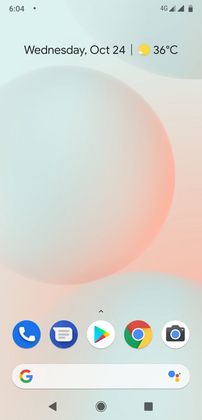A screenshot of a smartphone screen is prominently displayed. 

**Top Section:**
- **Upper Left Corner:** The time is displayed as "6:04" in black font.
- **Upper Right Corner:** Various status icons are visible, including the battery icon, the Wi-Fi signal icon, and the "4G" indicator, all in black font.
- **Upper Center:** The date is shown as "Wednesday, October 24th" followed by a pipe symbol. To the right of the pipe symbol, there’s a temperature reading of "36°C" accompanied by a sun icon.

**Middle Section:**
Below the top information, there is a significant blank area before reaching the bottom portion of the screen.

**Bottom Section:**
- **Icon Row:** There are five clickable icons arranged horizontally:
  1. **Telephone Icon:** Represents the phone application.
  2. **Chat Icon:** Likely for messaging or a communication app.
  3. **Google Play Icon:** Directs to the Google Play Store.
  4. **Google Icon:** Possibly for the main Google app.
  5. **Camera Icon:** For the camera application.
- **Google Search Field:** Just below the icon row, featuring the Google logo ("G") and a search field for user input.
- **Navigation Bar:** At the very bottom, there are three navigation options:
  1. **Left Triangle:** Points left, used to navigate back to the previous screen.
  2. **Circle:** Located in the center, likely the home button.
  3. **Square:** Positioned to the right, for accessing the app switcher.

This detailed description captures all the observable elements on the smartphone screen, providing a clear and thorough understanding of the display.